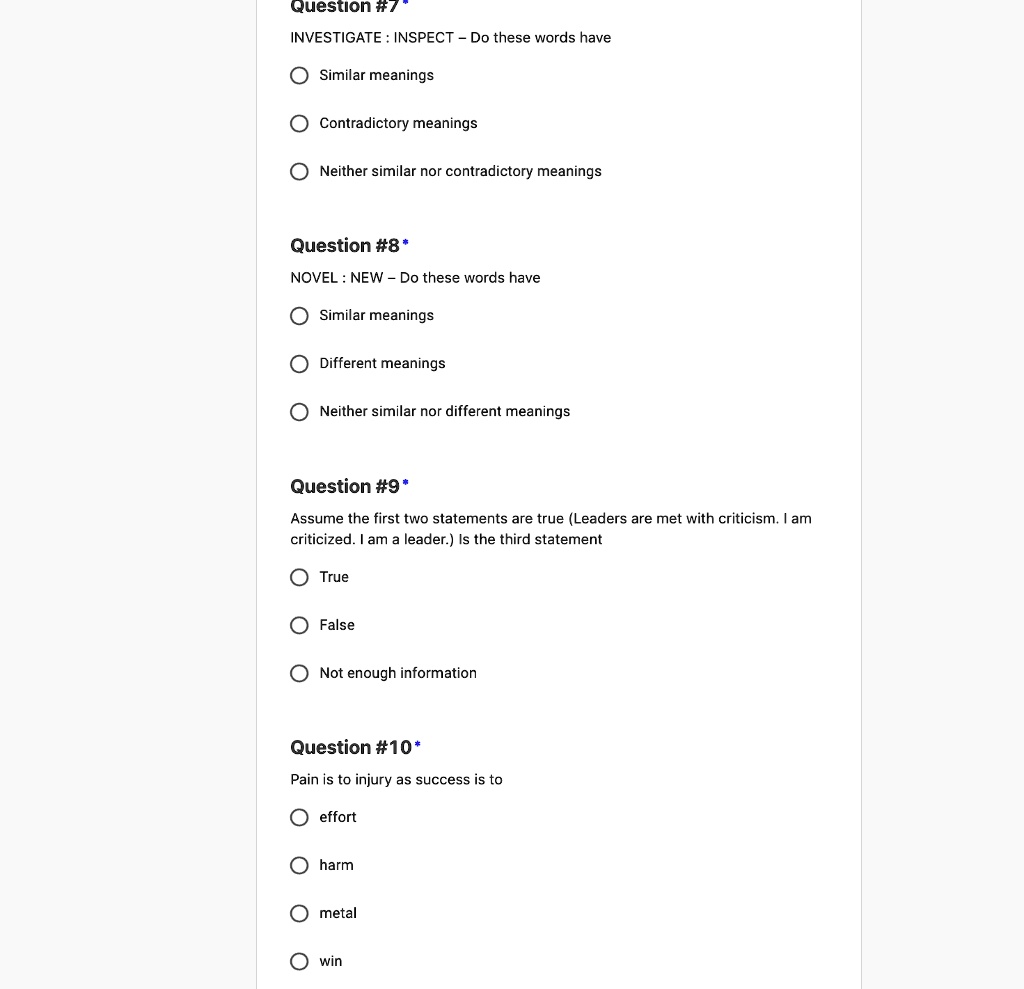This screenshot captures a portion of what appears to be a survey, quiz, or questionnaire featuring a white background with black text. The segment begins with "Question 7," highlighted in bold black text, followed by a series of standard black text queries. The query reads: 

"Investigate: Inspect - Do these words have:
- Similar meanings
- Contradictory meanings
- Neither similar nor contradictory meanings"

Subsequently, "Question 8" is also denoted in bold, followed by this query:

"Novel: New - Do these words have:
- Similar meanings
- Different meanings
- Neither similar nor different meanings"

Following the same format, "Question 9" in bold presents a logic statement and associated options:

"Assume the first two statements are true: 
- Leaders are met with criticism
- I am criticized
- I am a leader

Is the third statement:
- True
- False
- Not enough information"

Finally, "Question 10" relates to analogies, formatted similarly:

"Pain is to injury as success is to:
- Effort
- Harm
- Medal
- Win"

Each question and potential answer is presented with unbulleted bullet points beside them for response options.